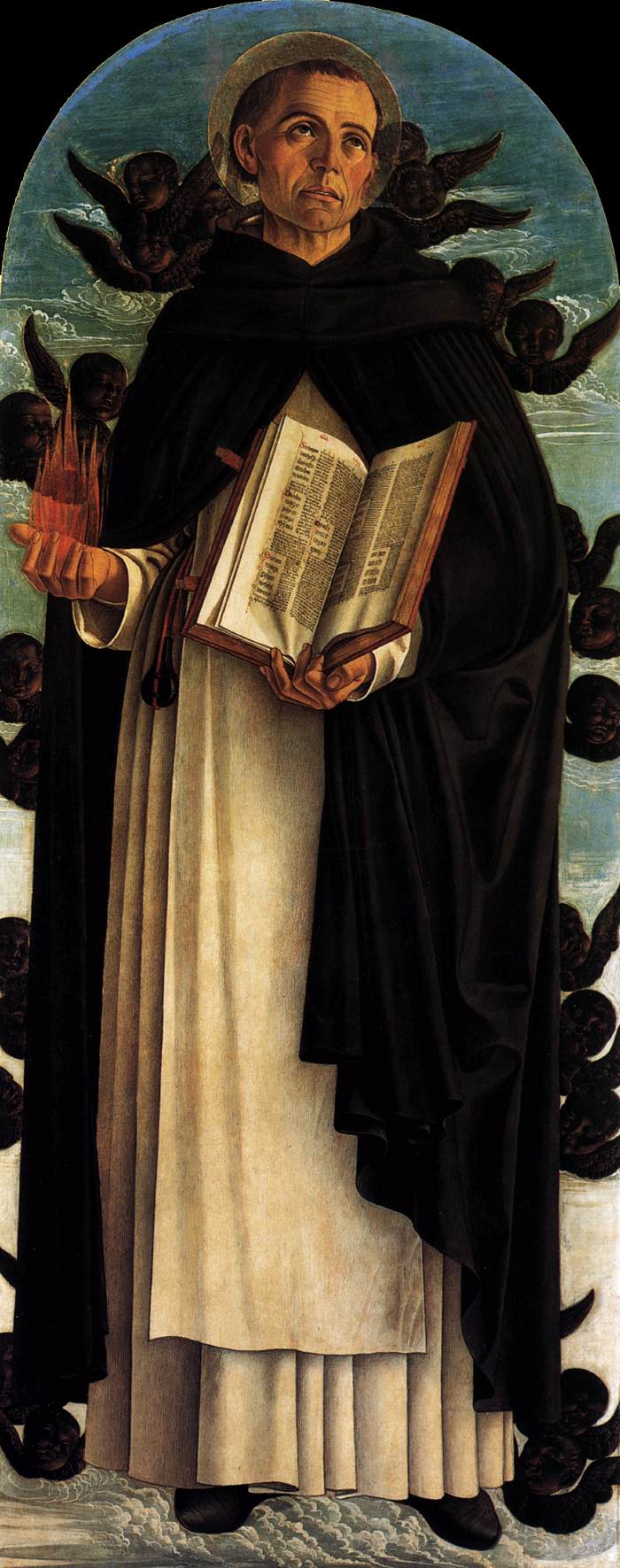The painting depicts an older priest or monk, characterized by his white robes that extend to his feet and a black cape draped around his shoulders and neck. His head is adorned with a halo, typical of many Catholic artworks, and his distinct tancha haircut. The priest is holding an open Bible facing outward, with visible text on the page. His pose conveys a pious demeanor as he gazes upward. The scene is set against a backdrop of a blue sky and clouds, with the bottom of his robe appearing creased like a curtain. Surrounding him are numerous angelic figures, depicted as cherubic heads with wings, some hovering by his shoulders and others extending down to his feet, seemingly supporting or elevating him. The overall composition gives an impression of ascension or divine support.